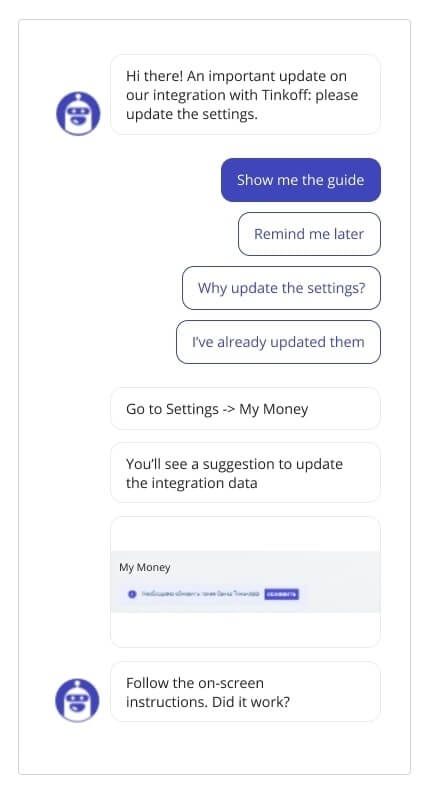A detailed caption for the image could be:

"This online screen image features a prominent notification banner at the top, stating 'Hi there, an important update on our integration with Tinkoff. Please update the settings.' Below this, a selection of tabs is displayed, the first of which is highlighted in blue and reads 'Show me the guide.' Following this, there is a sequence of banners that say 'Remind me later,' 'Why update the settings,' and 'I've already updated them.' Further down, text instructs users to 'Go to settings' with a right-pointing arrow leading to the words 'My Money.' Underneath, it states, 'You'll see a suggestion to update the integration data.' Another visible light banner box is labeled 'My Money,' though it contains text that is too small to read. At the very bottom of the screen, there is a circular systems icon resembling a robot head, accompanied by the message 'Follow the on-screen instructions.'"